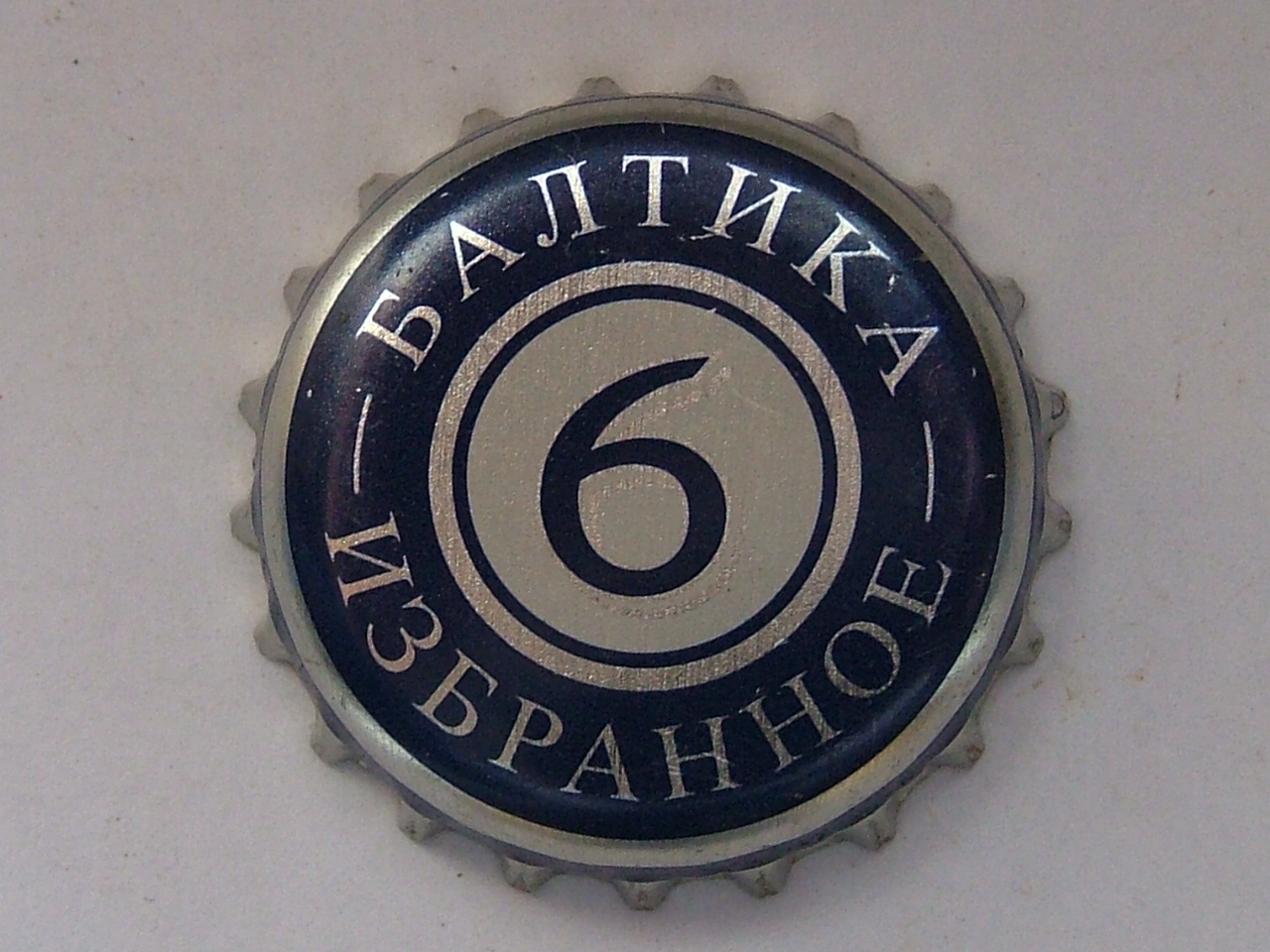The image showcases a close-up of a metal bottle cap resting on a slightly off-white countertop. The cap itself, although modern, mimics the vintage style and features a silver rim with a series of concentric circles. The innermost circle is a solid silver background with a large navy blue number six at its center, reminiscent of a billiard ball design. Surrounding this central circle is a thinner silver band, followed by a prominent navy blue band that contains text in what appears to be Russian, curving around both the top and bottom halves of the cap. The cap's metallic surface shows minor scratches, likely from being pried off the bottle. Overall, the bottle cap retains a clean and unblemished appearance.